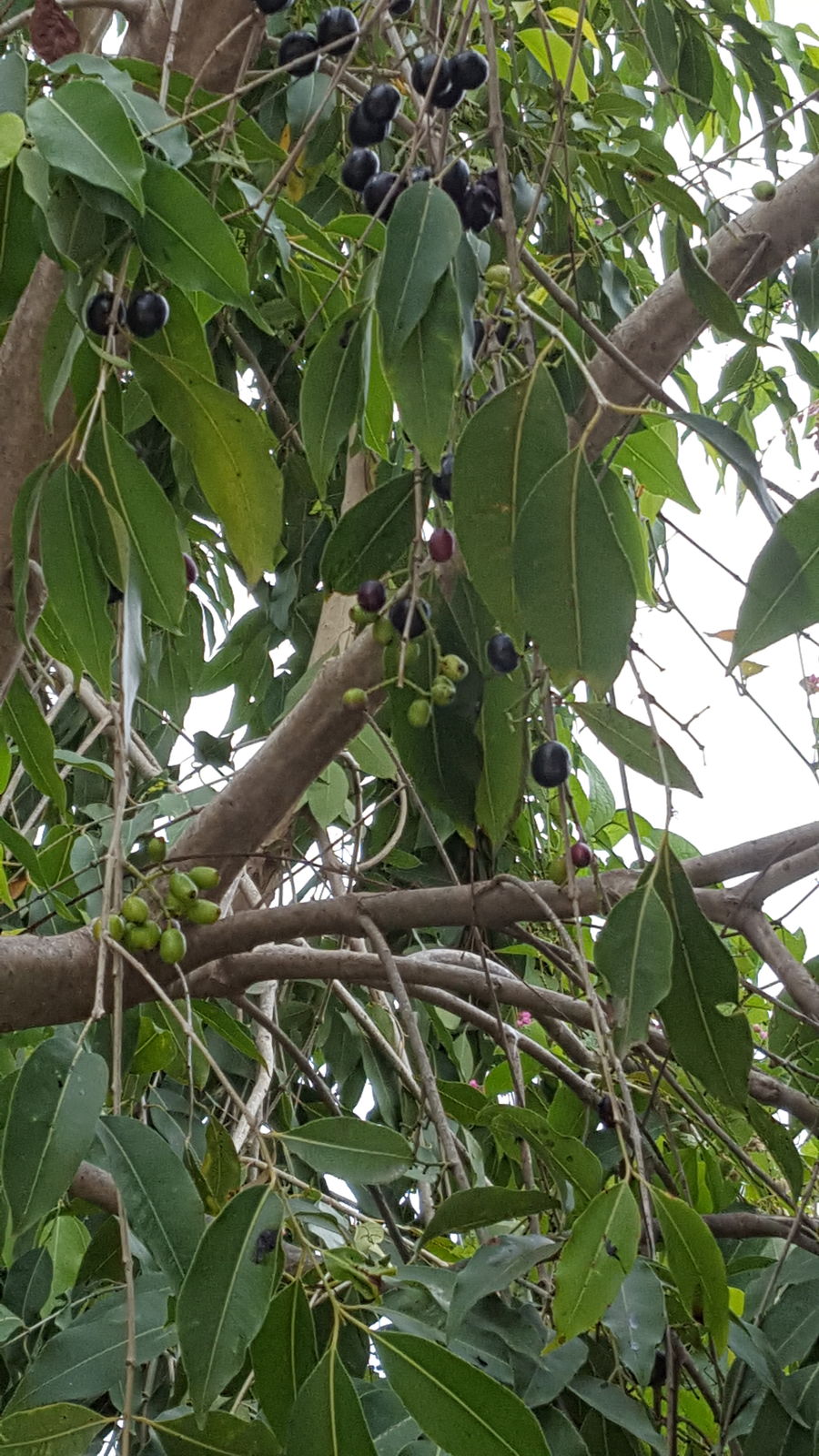This is a detailed photograph of a wild black cherry tree (Prunus serotina), commonly found throughout the southeastern United States, taken from the ground looking up into the branches. The image captures the tree at a stage where it has already flowered and transitioned to fruit-bearing, showcasing both green unripe and tiny black ripe cherries, each about half an inch in diameter. The tree's light brown to light gray branches extend vertically and diagonally, with some branches flowing horizontally and downwards. The branches are densely adorned with typical cherry leaves, which are oblong with a pronounced central stripe. The foliage appears in shades of lime to forest green. The background features a completely overcast, cloudy white sky, emphasizing the detailed and concentrated foliage and fruit. This photograph serves as an excellent identification image for the black cherry species, visually focusing on the characteristic leaves and small fruits.